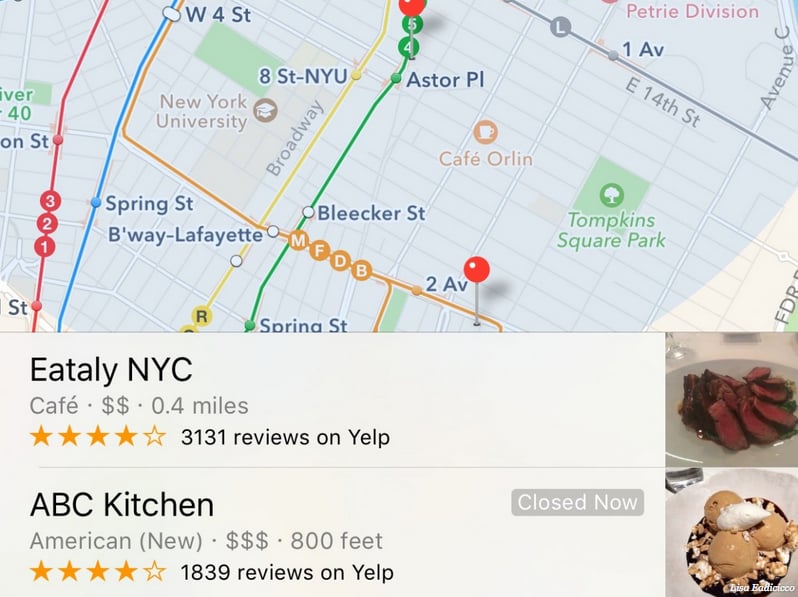This is a screenshot of a digital map that appears to show parts of Tompkins Square Park and Bleecker Street, suggesting a location in New York City, despite a misattribution to London. Highlighted on the map are several pins and numbers indicating points of interest, specifically restaurants.

Prominently featured is Eataly NYC Cafe, marked with a $2 sign symbolizing moderate pricing. It is located 0.4 miles from the current location and boasts a rating of four stars based on Yelp reviews. The imagery associated with Eataly NYC Cafe depicts a succulent medium-rare steak, suggesting an appetizing dining option.

Another highlighted establishment is ABC Kitchen, categorized as an American restaurant. Despite an expensive pricing marked by three $ signs, it maintains a strong four-star rating from 1,839 reviews, although it is currently closed. The visual representation for ABC Kitchen includes hamburger buns and an eclectic assortment of items on the plate, contrasting with the more traditional dish shown for Eataly NYC.